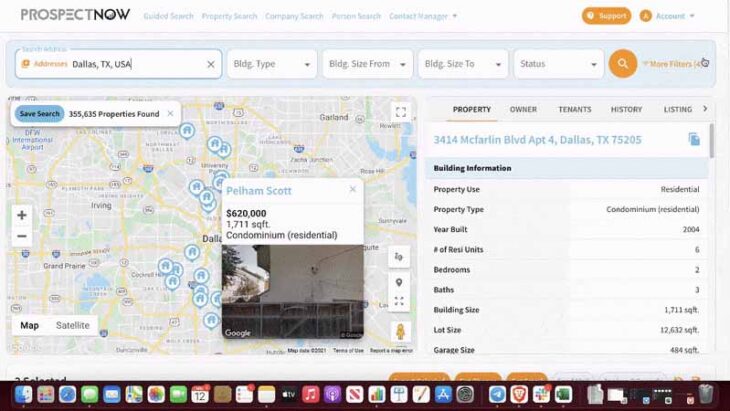The screenshot showcases the Prospect Now website running on macOS, as evidenced by the taskbar at the bottom filled with various application icons. The main content on the screen features a detailed map view, typical of real estate websites, with multiple clickable location markers. The user has hovered over a specific property listed as "Pelham Scott," a condominium valued at $620,000, and measuring 1,700 square feet. The image displayed for Pelham Scott is rather plain, depicting a wall and a fence. On the right side, an information pane provides further details about the property: it is designated for residential use, was built before a specified year, contains six residential units, has two bedrooms and three bathrooms, with a building size of 1,700 square feet and a lot size of 12,632 square feet. This suggests the property could either be an expensive single-family house or an affordable apartment building.